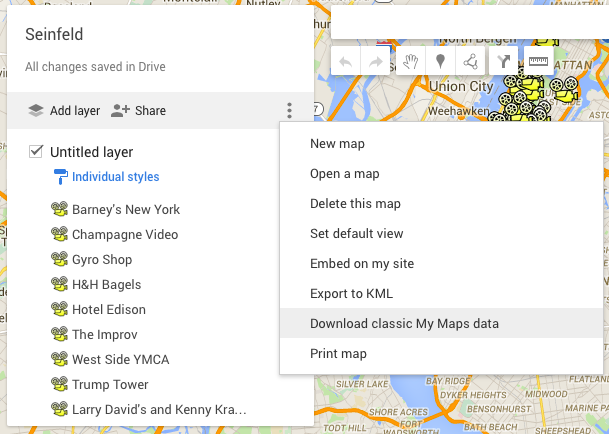In this image, we observe a screenshot of a digital map interface, showcasing a variety of on-screen textual elements and map-related features. The map platform allows for the addition of layers and offers functionality such as sharing, saving changes to the cloud (Drive), and customizing individual styles. 

The "untitled layer" is highlighted, and a series of location markers are visible, identifying notable places such as Barneys New York, Champagne Video, Gyroshop, H&H Bagels, Hotel Edison, The Improv, Westside YMCA, and Trump Tower. Additionally, Larry David's name is paired with 'Kenny,' likely referring to a specific point of interest on the map.

The interface includes several command options: creating a new map, opening an existing map, deleting the current map, saving the default view, embedding the map on a website, exposing the map data to KML format, downloading classic map data, and printing the map.

In the background of the screen, names of various cities and neighborhoods can be seen, including Union City, Weehawken, Bentonhurst, Bath Beach, Dyker Heights, Bay Ridge, Silver Lake, and Shaw Acres, indicating the geographical scope of the map displayed.